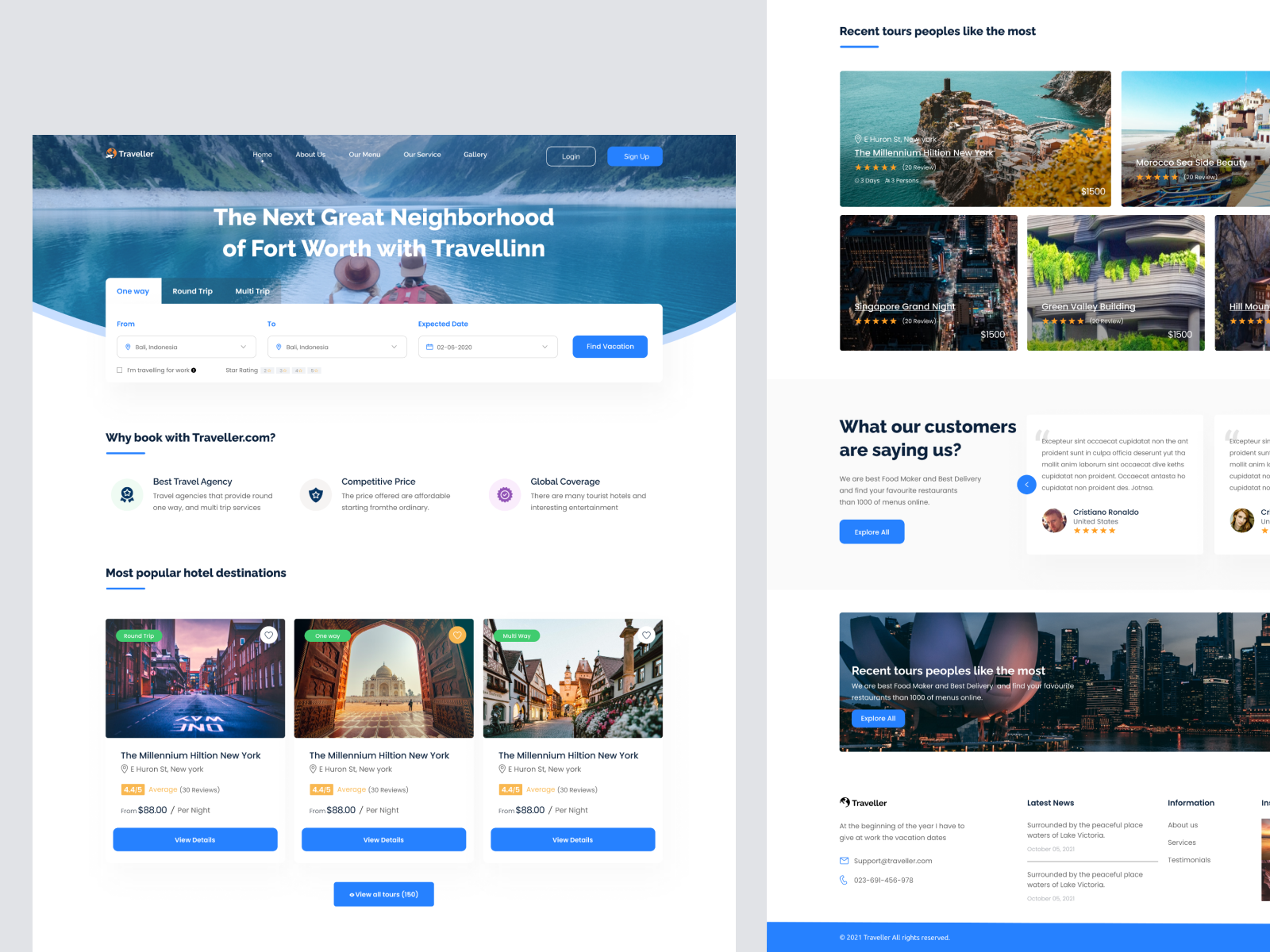### Detailed Description of the Web Page Image

The web page is divided into two sections, with each section showcasing different content.

#### Left Section:
- **Borders and Colors:**
  - The left section has a distinctive gray border outlining its left, right, and top edges.
- **Blue Banner:**
  - Just below the gray border, there is a blue banner.
  - The blue banner contains white text stating, "The Next Great Neighborhood of Fort Worth with Travel Land."
- **Visual Elements:**
  - Within the blue banner, there is an image showing the back of two people wearing hats.
- **Search Functionality:**
  - Below the blue section, there is a white background featuring three search boxes where users can enter information.
  - Adjacent to the search boxes is a blue button designed for users to click and proceed.
  
- **Informative Text:**
  - Below the search boxes, in bold black letters, it says "WhyBookWithTraveler.com."
  - There are three highlighted informational categories:
    1. Best Travel Agency
    2. Competitive Price
    3. Global Coverage 
- **Popular Destinations:**
  - Further down, there is a section titled "Most Popular Hotel Destinations."
  - This includes three clickable images, each with price details underneath, though the text appears small and somewhat difficult to read.

#### Right Section:
- **Top Header:**
  - The top of the right section reads, "Recent Tours People Like Most."
- **Tour Images and Ratings:**
  - Below this header, there are four images, each accompanied by ratings. However, the text associated with these ratings is very small and hard to read.
- **Customer Testimonials:**
  - Beneath the images, another segment in bold black letters states, "What Our Customers Are Saying to Us."
  - This section contains customer feedback, but like other parts, the text is small and may be challenging to read.

This detailed description provides a comprehensive overview of the layout, colors, images, and key text segments of the web page as described in the voice caption.